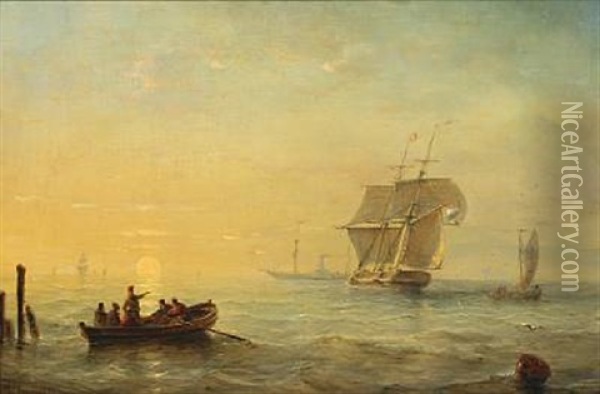This detailed painting, possibly a postcard, titled "NiceArtGallery.com" along the right-hand side, captures a historical maritime scene set during the dramatic light of either sunrise or sunset. The foreground features a small rowboat carrying five men, one of whom is standing and pointing towards a large schooner with sails. The schooner appears battle-worn and slightly tilted, suggesting it has recently been in conflict. The setting is a bustling harbor or lake with at least three or four boats visible. The water, painted in beautiful hues of green, gray, and touches of yellow, looks choppy. The sky transitions from an orange-yellow near the horizon to a bluish tint at the top, adding to the overall ambiance of the painting. Large circular wooden posts are also visible, typically used for docking, indicating the men are departing from a shore. The scene is enveloped in a harmonious, yet poignant light, accentuating the historic and adventurous nature of the image.